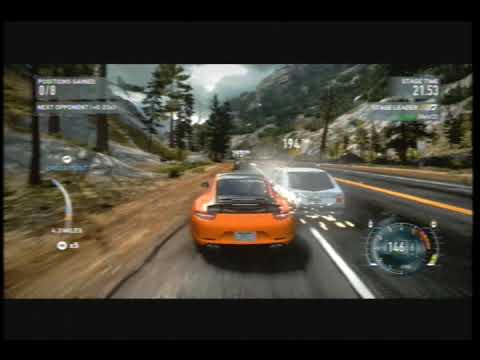The image is a blurry screenshot from a racing game, framed by thin black bars at the top and bottom, with larger dark grey bars inside. At the center of the frame, an orange sports car, viewed from a third-person perspective, speeds down a winding country road flanked by mountains and pine trees. To the right of the orange car, a white or silver hatchback car appears to collide with it, creating yellow sparks between the two vehicles. The paved road features the standard orange and yellow lines, and a speedometer in the bottom right corner reads 146. Additional icons and measurements, including gear and possible attack time, are displayed along the top right and left side panels. A house is faintly visible in the background to the left.